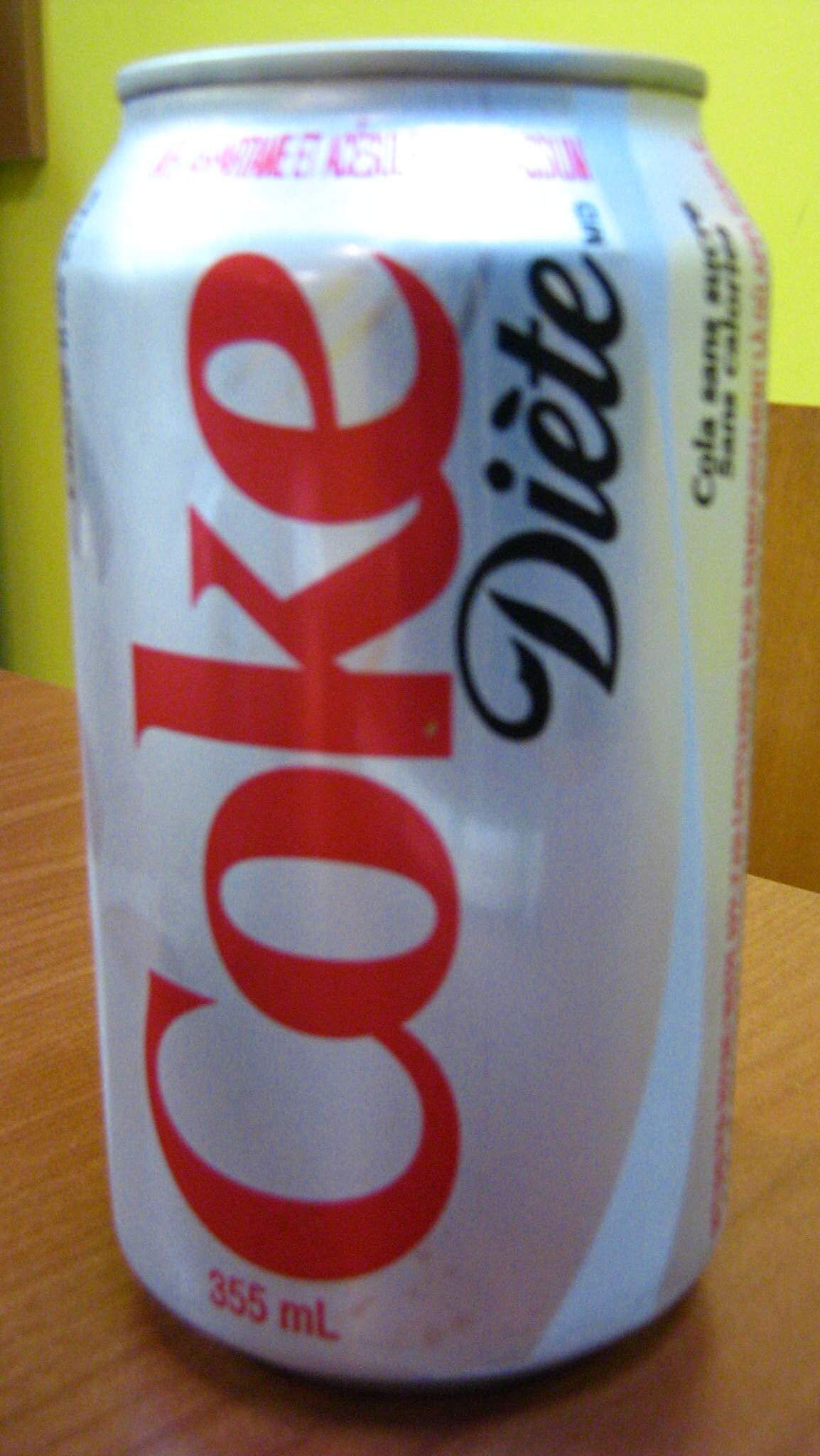This image features a silver can of Diet Coke positioned on a brown, wood-textured surface. The photograph is notably blurry, with low resolution, affecting the clarity and details of the scene. The can lies horizontally, displaying the word "Coke" written in red and located sideways, accompanied by "Diet" inscribed below in black. Underneath, the number "355" is visible. In the background, the wall is painted a yellow hue, providing contrast. Additionally, a dark brown object, partially cut off and unidentifiable, is seen in the top left corner of the image.